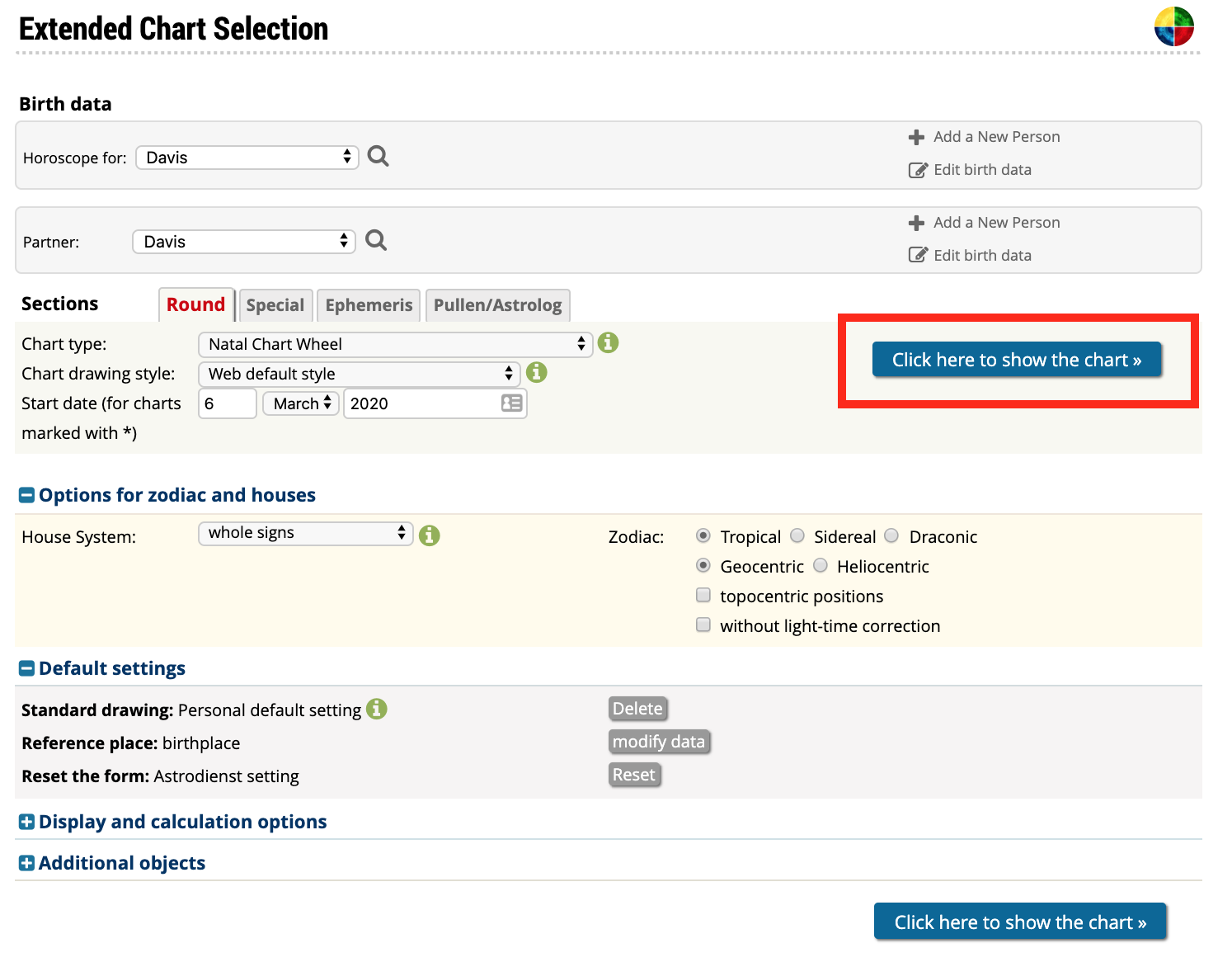In this image, we are looking at a screenshot displaying an interface related to astrology. In the upper left corner of the image, there is black bold text reading "Extended Chart Selection". Below this text is the label "Birth Date" and the heading "Horoscope for Davis Partner Davis."

To the right of these headings, there are several small boxes labeled "Round," "Special," "Ephemeris," "Pollen," and "Astrologe," which seem to be different sections of the chart selection interface. Further right, the text indicates "Chart Type" and specifies "Natal Chart Wheel." The "Chart Drawing Style" is listed as "Web Default Style."

The starting date for the chart shown is marked as March 6, 2020. Below this primary information, the next section on the screen reads "Options for Zodiac and Houses." Directly beneath this, there is a bar under the term "House System," specifying it as "Whole Signs."

The visible options for Zodiac include "Tropical," "Side Wheel," "Draconic," "Geocentric," "Heliocentric," and "Topocentric Positions without Light Time Correction." 

Lastly, there are sections for "Default Settings," "Display and Calculation Options," and "Additional Objects," presumably providing further customization for the astrological charts.